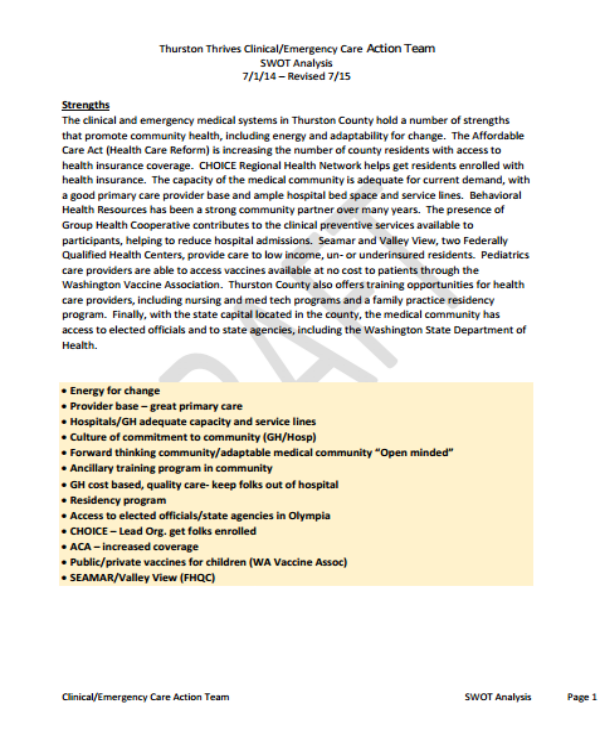This image is a detailed screenshot of a draft document, indicated by the faint diagonal watermark reading "DRAFT" across the background. The watermark's letters "A-F-T" and part of an "R" are clearly visible. The document's primary background is white with black text, but the lower third features a tan-colored background also with black text, which partially conceals the rest of the watermark text.

Centered at the top, the document title reads "Thurston Thrives Clinical/Emergency Care Action Team" followed by the heading "SWOT Analysis" and the date of revision. Below this, the section titled "Strengths" is highlighted in bold and underlined text, leading into a substantial paragraph. The introductory sentence of this paragraph states, "The clinical and emergency medical systems in Thurston County hold a number of strengths that promote community health, including energy and adaptability for change." It also mentions, "The Affordable Care Act is increasing the number of county residents with access to health insurance coverage."

In the tan-colored section, there is a list of bullet points summarizing the key points from the preceding paragraph. The document thus appears to be a structured and detailed analysis focused on the strengths of clinical and emergency care systems within Thurston County, offering insights on community health improvements and insurance coverage enhancements under the Affordable Care Act.